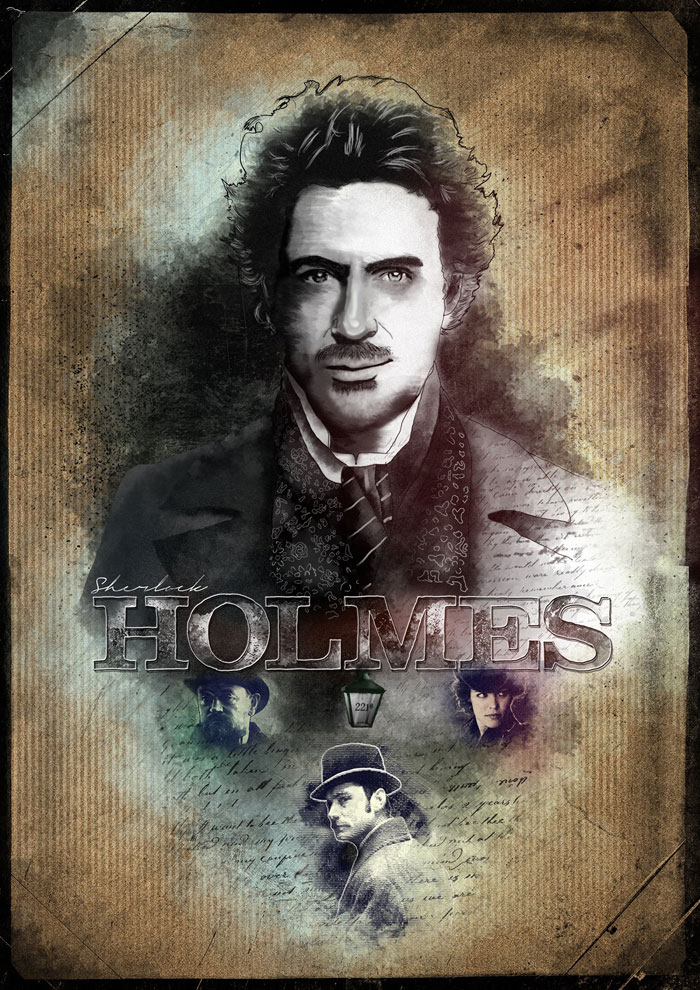The image is a horizontally aligned advertisement poster for a Sherlock Holmes themed movie or show, evocative of vintage style yet likely produced in the last decade. The main focal point is a black and white bust of Sherlock Holmes himself, centrally positioned and illustrated in a stylistically filtered, almost hand-drawn manner. Holmes, depicted as a white male in his 30s with dark, bushy hair, pronounced eyebrows, a bushy mustache, and a small beard or goatee, exudes a mysterious, brooding look with a shadow cast on the left side of his face. He is adorned in a 1920s-style suit featuring wide notched lapels, a distinct striped tie, and a patterned trench coat.

The background is a textured, cardboard brown with soft vertical lines that enhance the vintage aesthetic. The poster prominently displays "Sherlock Holmes" across Holmes' chest in bold, shiny capital letters resembling Times New Roman font. Beneath this central figure are smaller, intricately detailed portraits of three other characters. To the left is a man with a bowler hat, a dark beard, and a black suit. To the right is a young Caucasian woman, possibly in her 20s, wearing a hat and appearing to look off to the right. Centrally placed between the letters "L" and "E" of 'Holmes' is another man seen from behind, his head slightly turned to reveal a worried expression and a fine mustache. He is dressed in a gray coat and a flatter-than-usual top hat. 

The overall design of the poster, with black edges fading into the distressed, ink-stained look of the characters, contributes to its vintage yet contemporary appeal, making it a visually compelling piece.